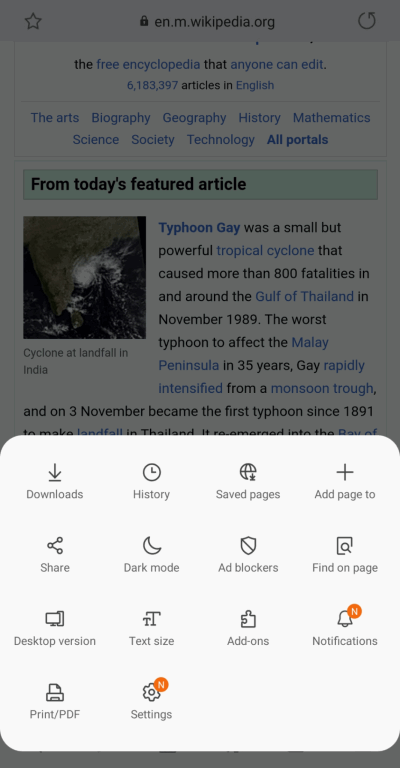This screenshot captures the mobile version of a Wikipedia page, specifically from en.m.wikipedia.org, the free encyclopedia that is open for public editing. The page prominently states that there are 6,183,397 articles available in English. Various categories such as the arts, biography, geography, history, mathematics, science, society, technology, and all portals are accessible from this page.

The screenshot highlights "Today's featured article" which describes Typhoon Gay. This tropical cyclone, noted for its small size but formidable power, resulted in over 800 fatalities in and around the Gulf of Thailand in November 1989. It stands as the most devastating typhoon to impact the Malay Peninsula in 35 years. The article details Typhoon Gay's rapid intensification from a monsoon, and its notable history-making event on November 3rd, 1989, when it became the first typhoon since 1891 to make landfall in Thailand. Unfortunately, the text abruptly ends here due to an overlay obstructing the remainder of the article.

This overlay is a white pop-up box presenting various option settings including downloads, history, saved pages, add to page, share, dark mode, ad blockers, find on page, desktop version, text size, add-ons, notifications, print/PDF, and settings. These options are visibly layered over part of the article, partially obscuring the content underneath.